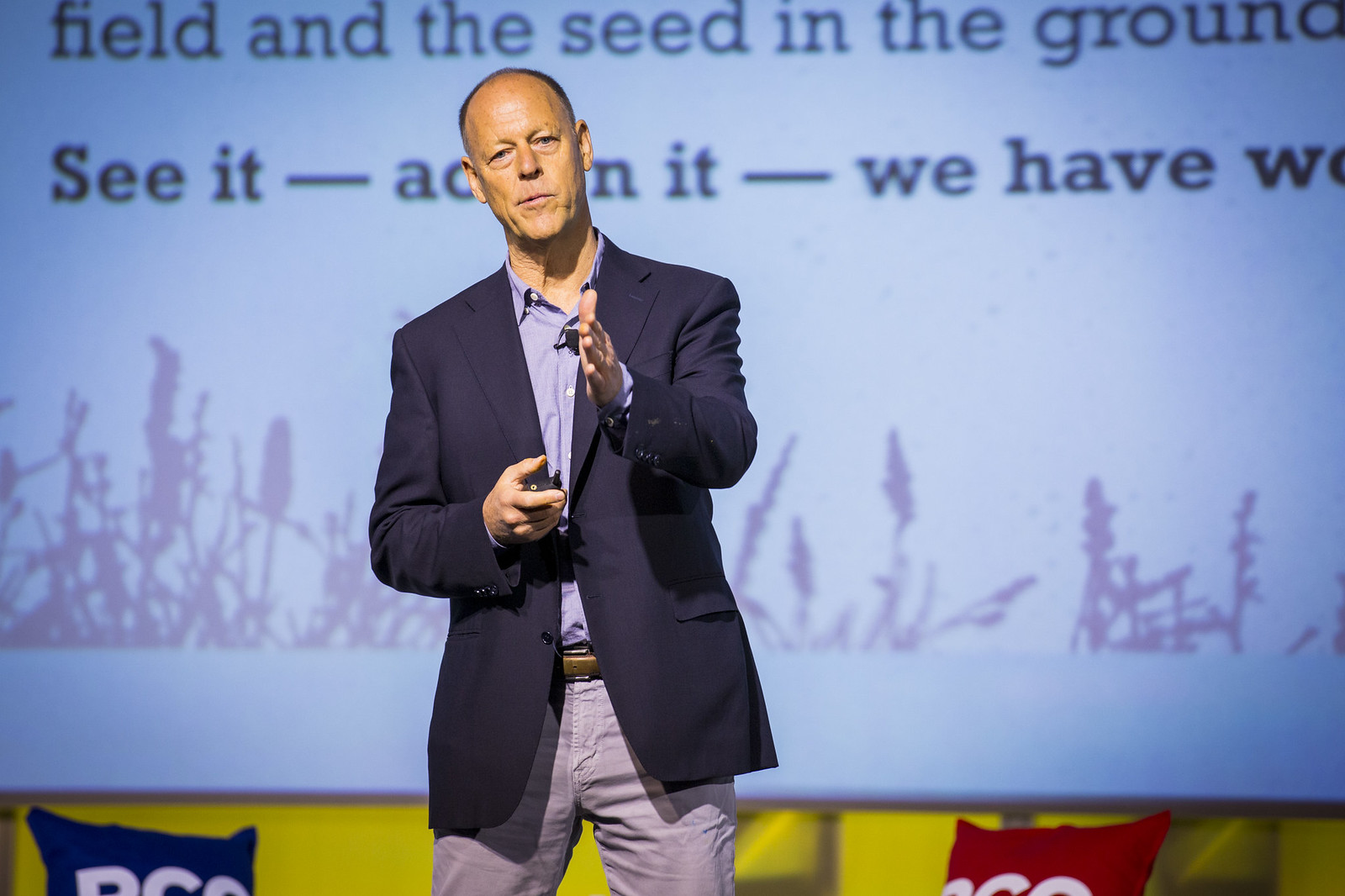The image features a Caucasian man, approximately 50 to 60 years old, mid-speech and gesturing passionately with his hand. He is dressed in business casual attire, wearing a navy blue jacket, a light blue shirt, stone-colored khakis, and a brown leather belt. The man's short dark hair is neatly shaved, and he is smirking slightly as he talks. He appears serious and engaged with his audience.

In the background, a large screen with partially visible text stands behind him, displaying the words, "Field and the seed in the ground, see it... we have." The background's dominant colors include light blue text on the screen and a yellow hue behind it. The words on the screen and the man's animated demeanor indicate he is in the middle of a presentation, likely using a remote to control the slides. The image captures both his intensity and the audience's mild amusement.